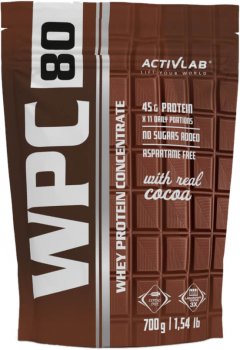This promotional image features Active Lab's Whey Protein Concentrate (WPC) 80, a specialized supplement powder designed for individuals looking to build muscle mass. The packaging is predominantly brown, evoking a rich, chocolatey flavor, reinforced by an overlaid chocolate bar graphic in the background. Prominently displayed on the left-hand side of the packaging, the product name "WPC 80" is written in large, bold white letters. Throughout the rest of the package, various white text details the nutritional benefits and key ingredients of the whey protein concentrate, providing essential information for potential consumers. The overall design effectively communicates the product’s muscle-building purpose and its delectable chocolate essence.